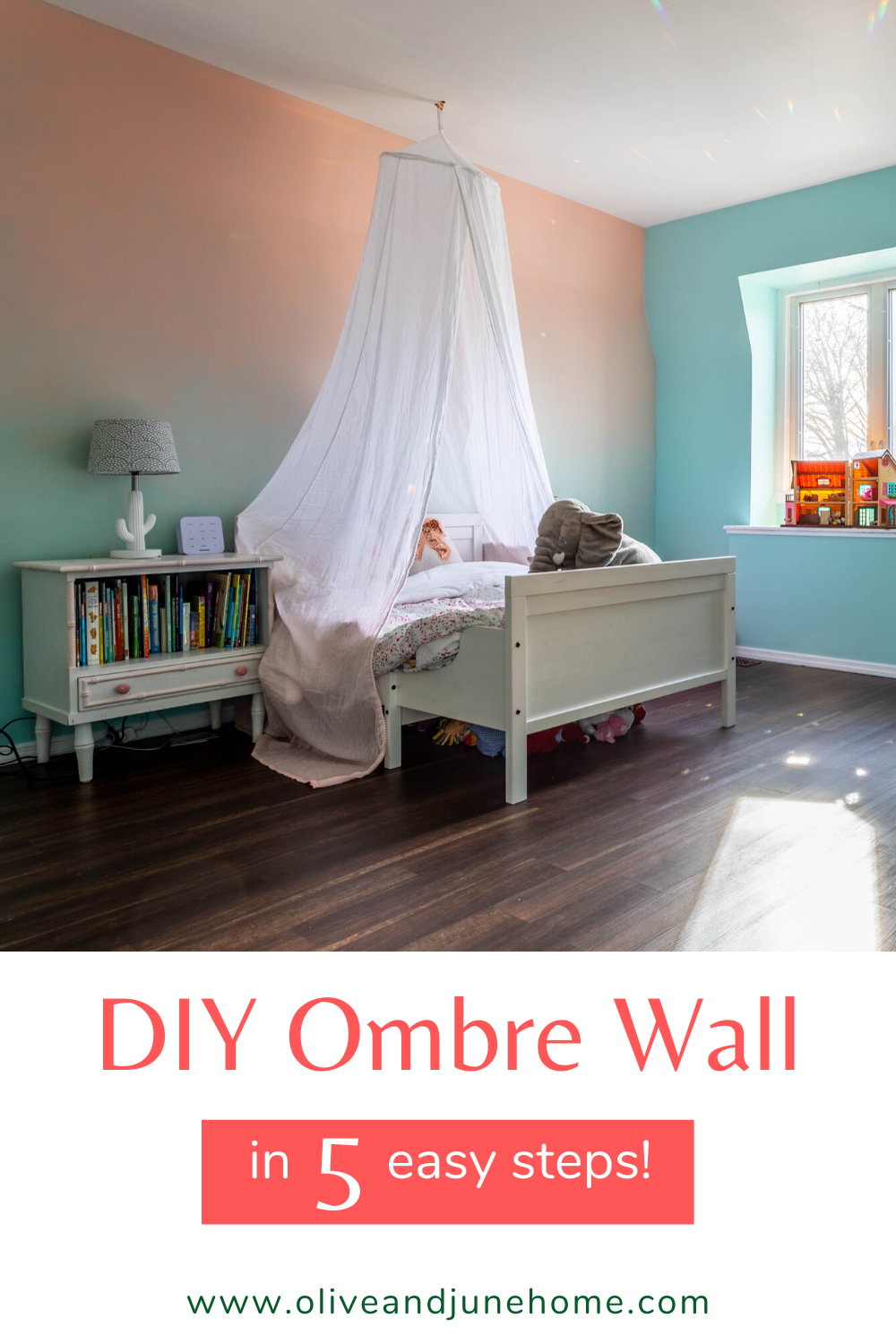The image is an advertisement for a DIY Ombre Wall project, presented in a format that layers a photograph of a bedroom over text. The bedroom features a unique wall design with a gradient ombre effect, transitioning from a pinkish hue at the top to a light blue-green at the bottom on the left-hand side, and light blue on the right-hand side. Central to the room is a white wooden bedframe, adorned with pillows and covered by a white net canopy hanging from the ceiling, giving it a tent-like appearance commonly used for protection against mosquitoes. The bed features brown and white pillows, and beneath it are some stuffed animals. 

To the immediate left of the bed is a wooden bookshelf, stocked with colorful children's books, a white alarm clock, and a distinctive white cactus-shaped lamp with a gray shade. To the right of the bed is a window with a shelf that holds a dollhouse. The room has a dark brown hardwood floor that reflects light, adding a warm ambiance to the space.

Below the photograph, on a white background, the text reads in a sequence of red and white fonts, “DIY Ombre Wall in Five Easy Steps," with the website www.oliveandjunehome.com displayed, directing viewers to further details.